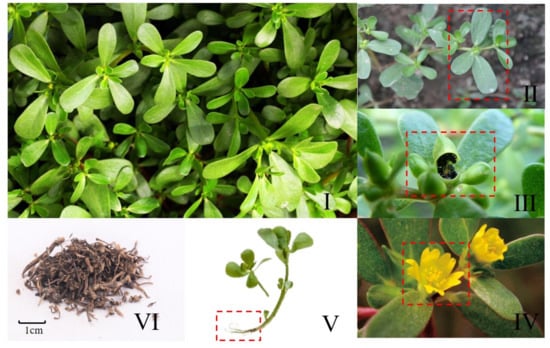The image is a detailed depiction of the progression stages of plant growth, divided into six segments marked by Roman numerals. In the largest segment, Roman numeral I (upper-left side), a dense cluster of small green plants dominates the view, showcasing the bustling life of the seedlings. On the upper-right side, marked by Roman numeral II, similar green plants can be seen growing from the soil, with a red dotted line box highlighting one specific plant. Below this, in segment III, there's a close-up view of a few plants, also with a red dotted line box encircling a particular plant.

In the fourth segment, marked by Roman numeral IV, a green plant with a prominent yellow flower is displayed, again bordered by a red dotted line box to draw attention. Segment V, located to the left of the fourth, presents a singular piece of the plant, focusing on the stem area where a red box is highlighting the lower part near the root. Finally, Roman numeral VI, situated to the far left at the bottom, shows an area with soil, annotated with the measurement “1cm” beneath it, possibly indicating the depth or scale of planting.

This intricate and methodical illustration provides a visual journey from the initial stages of sprouting through full bloom to the foundational soil, each phase meticulously outlined and highlighted for clarity.